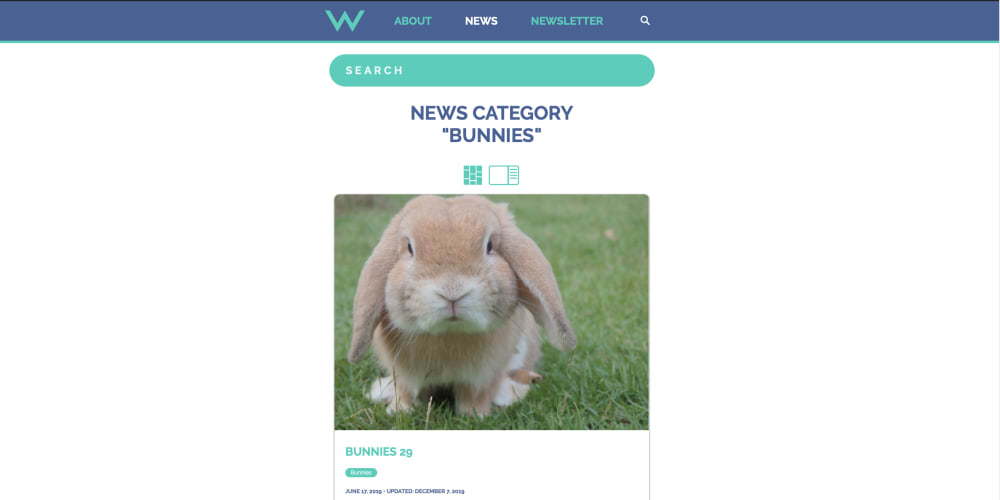This is a detailed screenshot of a modern, minimalist website. The website features a blue top bar with a centrally placed 'W' logo. Directly to the right of the logo are three navigation tabs labeled "About," "News," and "Newsletter." Adjacent to these tabs, there is a white magnifying glass icon indicating a search function. Below the top bar, there is an ovular, teal-colored search bar prominently displayed on a white background.

The main content of the page begins with a text heading that reads "News Category: 'Bunnies'." Below this heading, there are two buttons designed for changing the navigation style. The central focus of the page is an image of a bunny, and beneath this image, the text reads "Bunnies 29." 

There is additional text visible, which includes two date references: "June 17, 2019" and "Updated December 7, 2023," though the second date appears somewhat blurry and may alternatively be "December 7, 2019." The overall design of the website is characterized by its modern and simplistic aesthetic, emphasizing clean lines and a minimalistic approach.